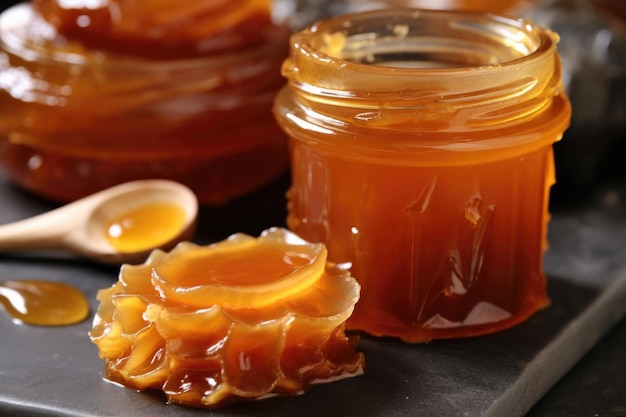This detailed photograph captures a close-up scene in a kitchen, centered around a jar that appears to contain honey, characterized by its amber, somewhat translucent liquid. The jar sits on a dark countertop, and next to it is a spoon coated with honey, suggesting a recent use. This spoon, along with a small blob of honey nearby, further emphasizes the jar's contents as honey. Adjacent to the jar, there is a piece of beeswax, matching the jar's mouth in size and possibly used to cover it. This beeswax is solid and waxy in texture, while having the same color as the honey. A tall, cake-like pastry in the background appears to have been drizzled with the honey, tying the elements together. The image, despite being bright and beautifully captured, suggests a somewhat messy but inviting kitchen scene focused on this luscious, golden honey.